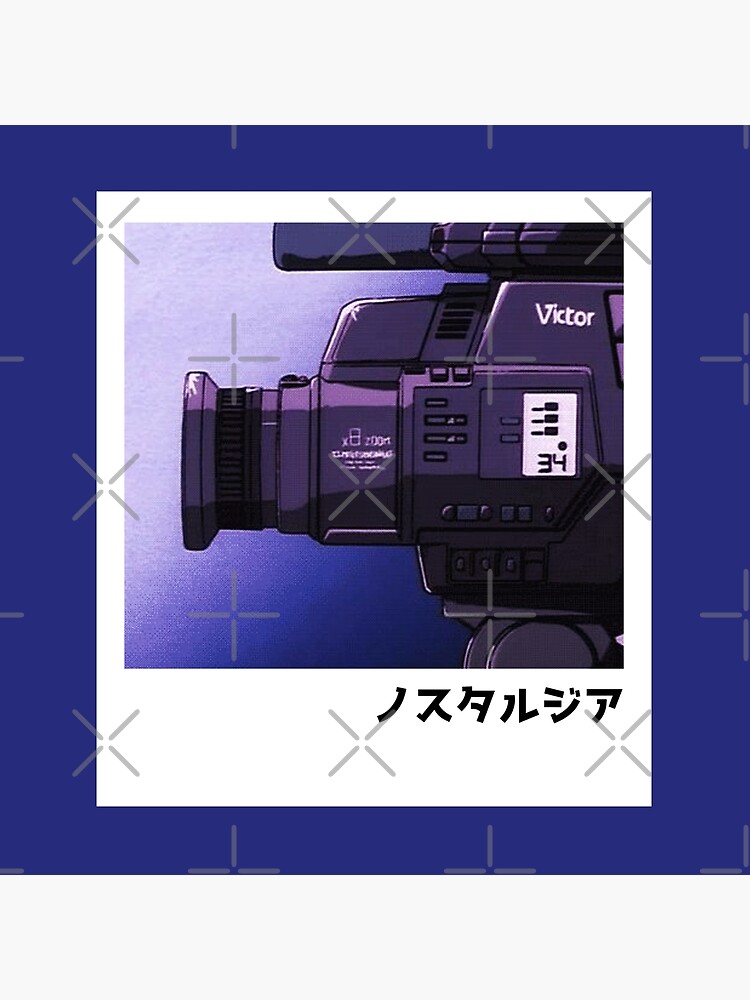The image is a cartoon-style depiction of a large, older-style video camera, specifically a Victor model. The overall background is a plain blue with cross patterns, transitioning to lighter shades of blue and white in some areas. Central to the image is a white Polaroid-style frame that contains the animated drawing of the camera. The camera is primarily black and purple with a detailed design featuring various buttons and dials, including a small white screen displaying the number 34. The brand name "Victor" is prominently displayed in white text on the upper right corner of the camera. Additionally, there are Japanese characters at the bottom of the Polaroid frame. The side view of the camera shows it looking to the left, adding a dynamic angle to the illustration. The entire image appears to be inspired by cartoon or anime aesthetics, accentuated by the watermark-like pattern of X's and crosses scattered across the scene.